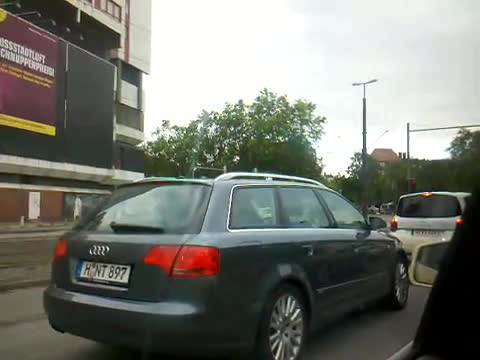In this atmospheric exterior shot, captured under the moody ambiance of natural, low dim lighting, the composition offers a compelling view through the driver's side window at a slight forward angle. The upper right portion of the frame showcases a stretch of somber, muted sky. To the left, the image includes a portion of a multi-story building, its facade only partially visible. Dominating the right side of the frame is a fragment of the car's rearview mirror, hinting at the perspective of the image taker. Adjacent, in the lane to the left, there is a dark gray hatchback sedan with a conspicuous, elongated, horizontally rectangular white license plate. The plate reads "H" followed by an obscured digit, and continues with "NT897," suggesting intrigue by the hidden character.